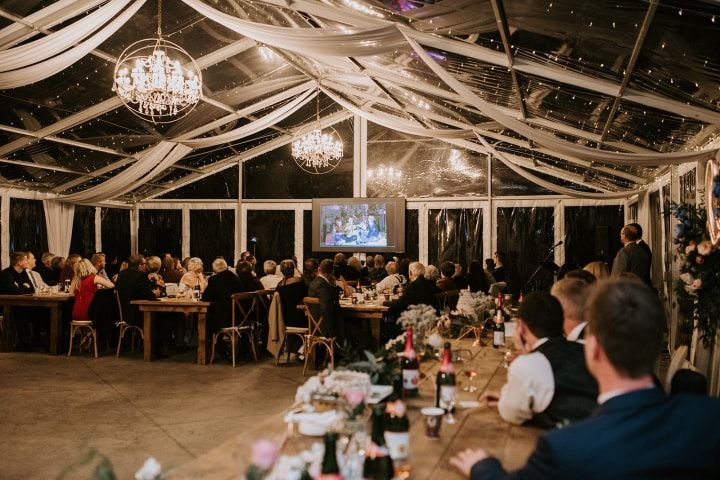This photograph captures an elegant wedding reception held inside a sophisticated, tent-like structure. The clear material of the tent allows natural light to filter in, beautifully illuminating the scene. Several long wooden tables, adorned with bottles of wine, teas, and floral arrangements, stretch across the venue, with people dressed in tuxedos, suits, and fancy dresses seated on either side. Their focus is directed towards a large screen displaying a sentimental slideshow, possibly featuring childhood photographs of the bride and groom. The ceiling is adorned with elaborate chandeliers and decorated with circular fabric strips, adding to the grandeur of the venue. The floor is paved with fine stone tiles, contributing to the overall luxurious ambiance.